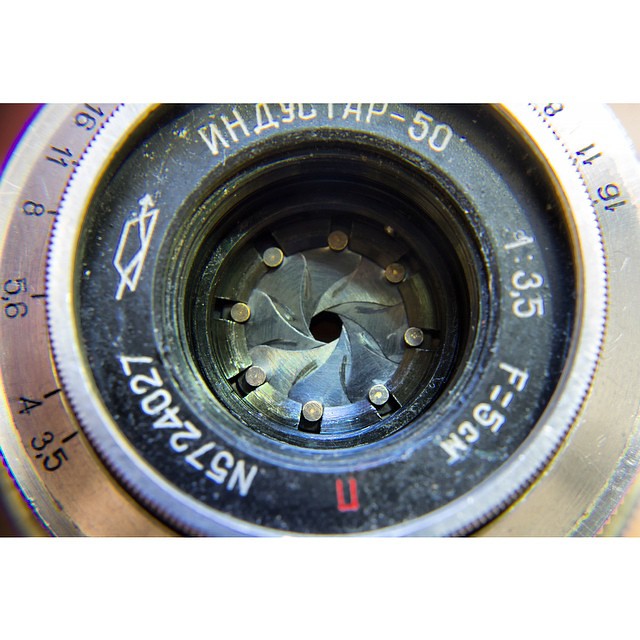This detailed close-up photograph captures the intricate components of an SLR camera lens. The central focus is on the round opening, almost closed, revealing the lens' aperture blades arranged in a circular, overlapping pattern. Encircling this centerpiece are eight visible rivets that secure the lens structure. The inner ring features a series of grooves and is marked with technical specifications such as "f=1:3.5" and "F=5cm." Moving outward, another metal band with numerals—ranging from 3.5 to 16—indicates the aperture settings, likely adjustable via a rotating dial adorned with ridges for better grip. This metallic ring transitions into a black outer circumference, printed with white lettering that appears etched into the surface. The golden or brassy outermost band, which also features numbers for additional settings or adjustments, completes the detailed engineering of this camera lens. The photograph extends beyond the edges of the image, emphasizing the grand scale and precision of this crucial photographic tool.